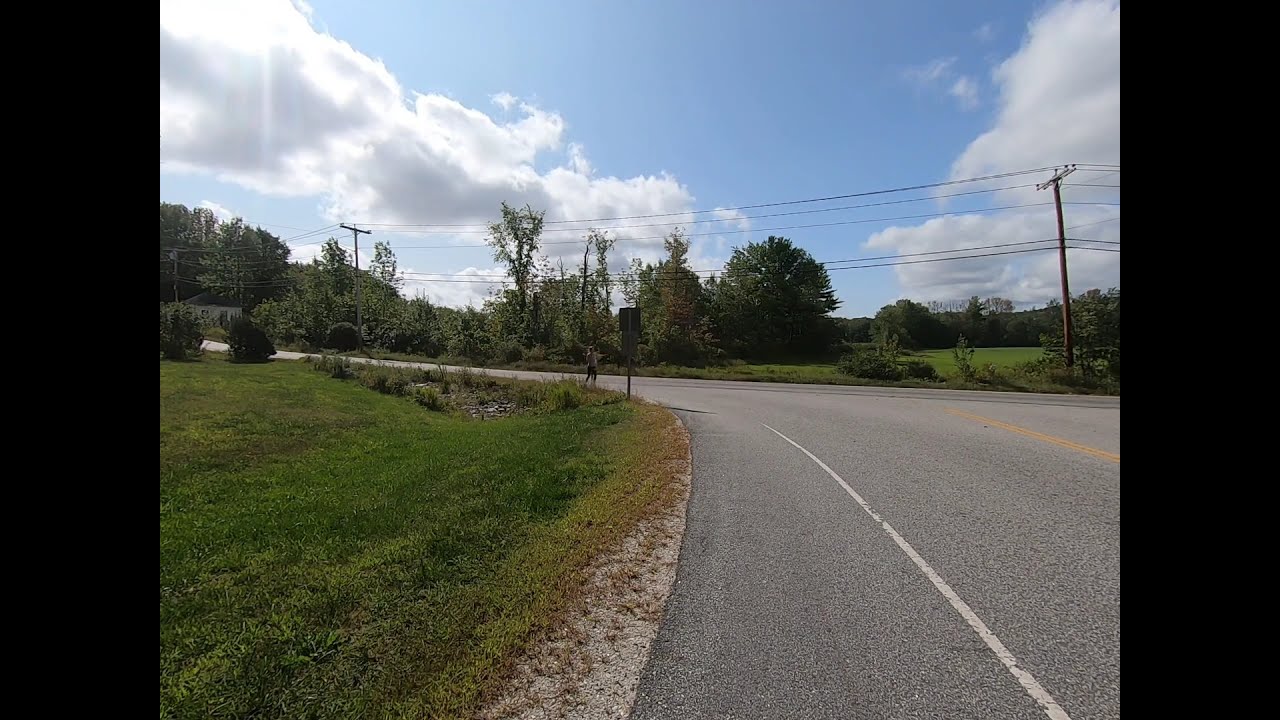The photograph depicts a curving road, likely a highway, where one road converges onto another. The road, made of light gray, bluish asphalt, dominates the lower right portion of the image and curves sharply to the left, tapering into the distance. To the left of the road lies a green grass area interspersed with patches of brown grass and a small ditch towards the center left. There is a distant, barely discernible pedestrian or hitchhiker near the curve of the road, standing close to a street sign, the back of which is visible.

Prominent in the scene are utility poles made of wood with power lines stretching horizontally across the image. The right side of the road is alongside some trees, while the left side features additional grassy areas with some dark green bushes. Above, the sky is mostly cloudy with a significant expanse of blue in the center, and areas where the clouds appear brighter and more illuminated, suggesting the position of the sun is to the left. The entire scene is framed within a rectangular format, with wide black bands on both sides, making the colored part of the photograph a bit wider than it is tall.